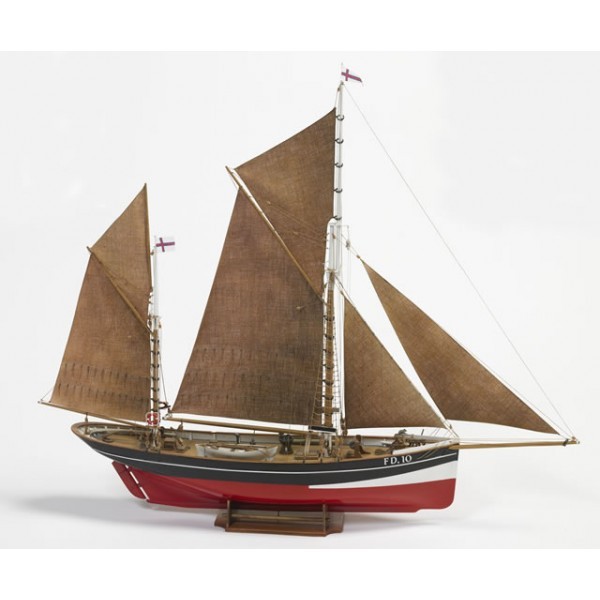This image features a detailed model of a sailboat set against an off-white background. The sailboat boasts a vibrant red hull at its base, transitioning to a smaller white, elongated triangle-shaped section towards the rear, and topped off with a black upper portion, distinguished by a single white stripe running its full length. Prominently displayed on the boat is the identifier "FD10." The boat is rigged with five aged canvas sails, mounted on two masts. Some sails are centrally located, while smaller ones are positioned both at the front (fore) and rear (aft) of the boat. The model is mounted on a brown wooden display stand. Additional details include a small flag bearing a red cross atop the mast. The interior of the boat is brown, with some hints of miniature elements that suggest a meticulous level of craftsmanship.